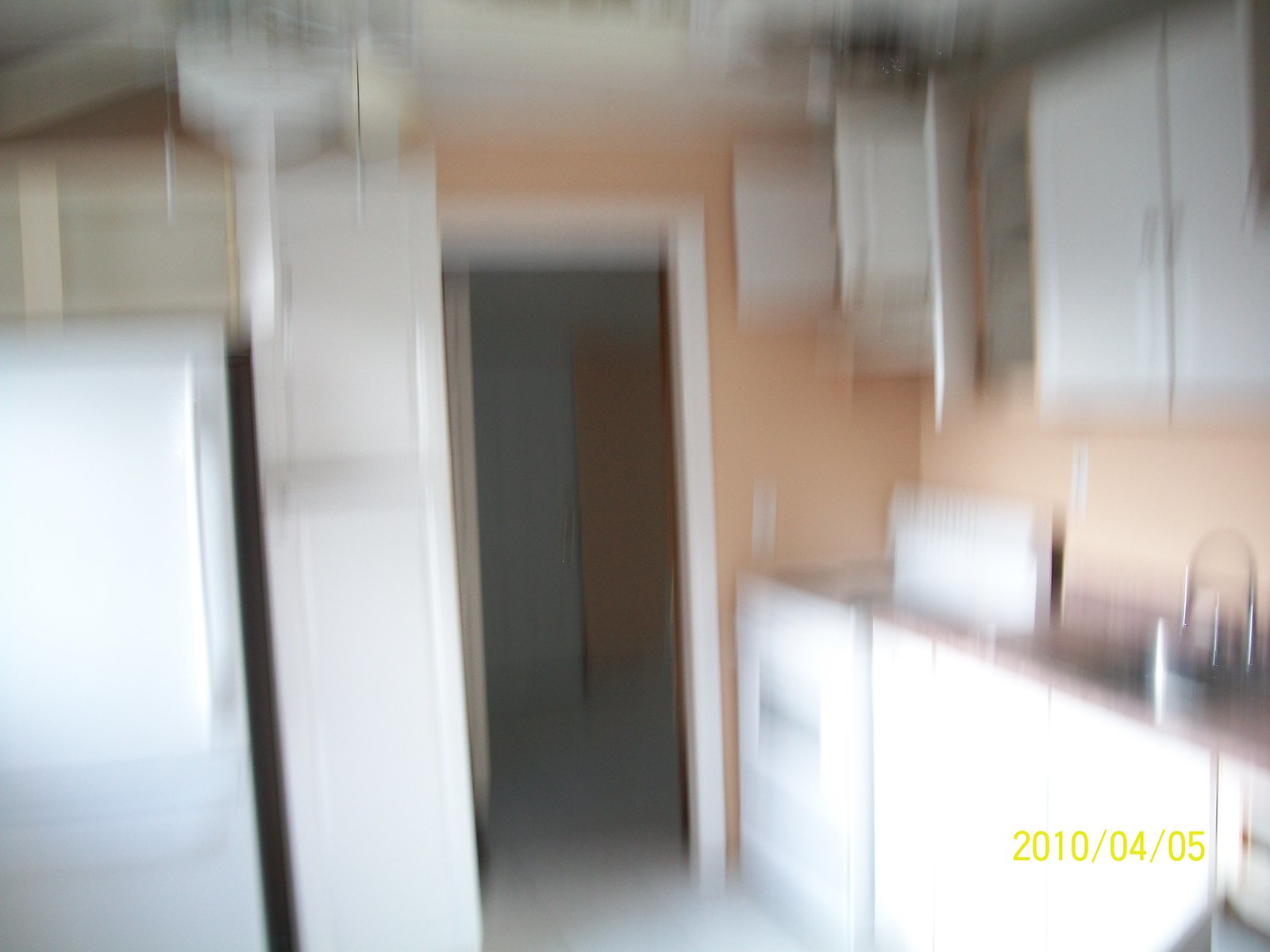The blurry image depicts a seemingly vacant kitchen with a distinct peach-colored wall, surrounded by white trim around the doorways. The kitchen is furnished with white cabinets, both upper and lower, some of which are open, revealing their empty interiors. Prominently placed in the room, the refrigerator, stove, and a tall white cabinet stand out against the peach walls. The countertop appears to be light beige or possible granite, though the image's blurriness makes it difficult to confirm. The silver sink faucet arches gracefully over the sink. Through the kitchen doorway, another unfurnished room is visible, casting shadowy impressions that add to the kitchen's abandoned feel.